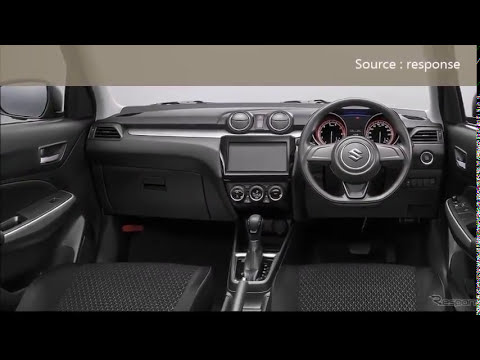The image depicts the interior of a vehicle, likely a Suzuki car, with the driver's side on the right, suggesting it is from a foreign country. The predominantly black interior features cloth seats and an array of electronic devices. An LED screen is centrally located on the console, and various knobs and dials are visible. The steering wheel, bearing an 'S' emblem, presumably for Suzuki, is on the right side. At the top of the interior, there's a text display that reads "source response," accompanied by light gray and almost white gray bars. The dashboard includes meters, an emergency brake, a gas pedal, a brake pedal, and a series of buttons, including a push-to-start button. The vehicle also has electronic doors, and visible mirrors can be seen through the windows.